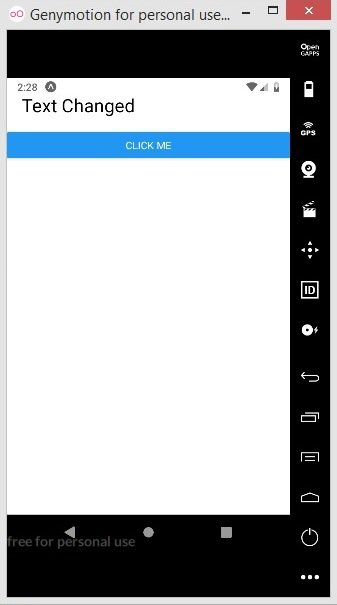Screenshot of an older mobile device using Genymotion emulator. The top of the emulator interface displays the text "Genymotion for personal use" alongside window control buttons, including maximize, minimize, and close options, suggesting it's running on a desktop operating system. The main screen of the emulator resembles the display of an Android device, featuring a black background adorned with a variety of app icons aligned on the right side. The app buttons typical of an Android interface are visible, including Back, Home, and Recent Apps buttons located at the bottom. The central focus of the screenshot is on an open application within the emulated Android device, displaying a simple user interface with the text "text changed, click me" and notable areas of white space.